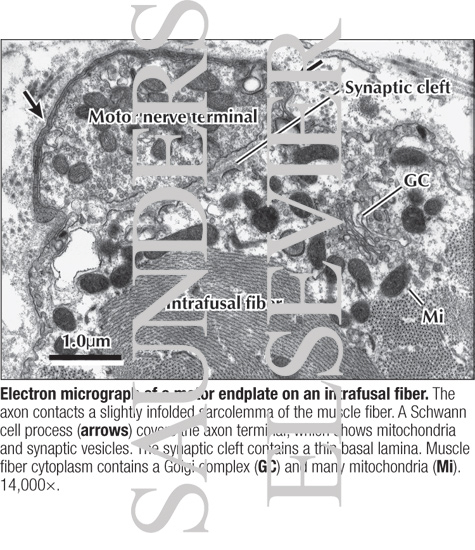This black and white electron microscope image depicts a motor end plate on an intrafusal muscle fiber. The landscape-oriented image shows intricate, swirling lines with dark, oval shapes scattered throughout, resembling cells. Various scientific terms and notations are labeled with blowout arrows pointing to specific areas of the image, such as the motor nerve terminal and the synaptic cleft. The bottom features a paragraph providing further details on the slide's subject. Overlaid vertically across the entire image is a watermark reading "Saunders Elsevier," indicative of the publishing house, which partially obscures some of the explanatory text.